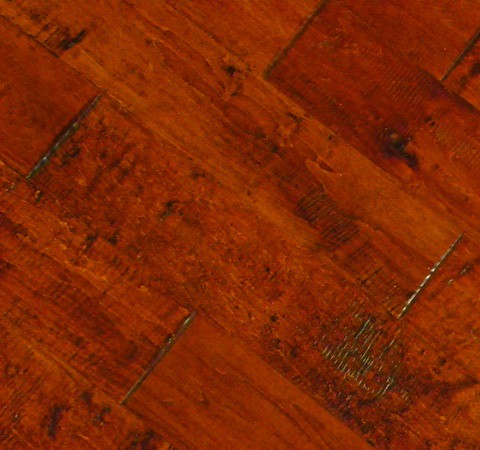This image captures a detailed view of a hardwood floor taken from an overhead perspective, emphasizing the variety in wood tones and textures. The scene reveals a carefully zoomed-in expanse of wooden planks that display a spectrum of browns, interspersed with shades of black and gray. The grains and veins of the wood are clearly visible, with darker veins concentrated at the bottom left, transitioning to gray veins in the middle and lighter veins at the top. The floor's finish is notably shiny, indicating a polished surface. At several points where the planks connect, the coloring darkens, hinting at aging or wear. Additionally, scattered across the floor are several metal objects. These appear to be narrow, cylindrical tools—potentially handles for branding irons or similar instruments—positioned in the upper left, center left, and mid-right areas of the floor. One particular item at the center right has a distinguishable design or symbol at its end. The overall setting is indoors, with the perspective suggesting the photo was taken from several feet above the floor, capturing both the intricate details of the wood and the mysterious metal objects.